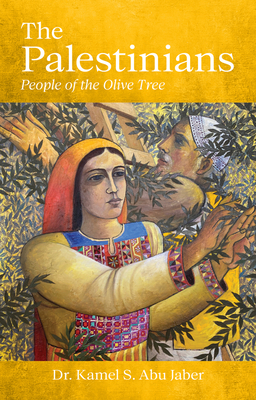The book cover predominantly features a golden yellow background with all text in white. At the top, the title reads, "The Palestinians," with a subtitle underneath stating, "People of the Olive Tree." At the bottom, the author's name, "Dr. Kamel S. Abu-Jabbar," is displayed. The centerpiece is a detailed drawing of a woman and a man interacting with an olive tree. The woman, dressed in a yellow headdress and a vibrant tunic-style dress featuring colors such as pink, blue, teal, and red, is running her hands through the tree's leaves. Her sleeves are yellow, matching her headdress. Behind her, slightly overlapping, is a man wearing a yellow garment with white pants and a light blue headdress, also engaging with the tree. Additionally, a wooden ladder is visible behind them, adding context to their interaction with the tree.